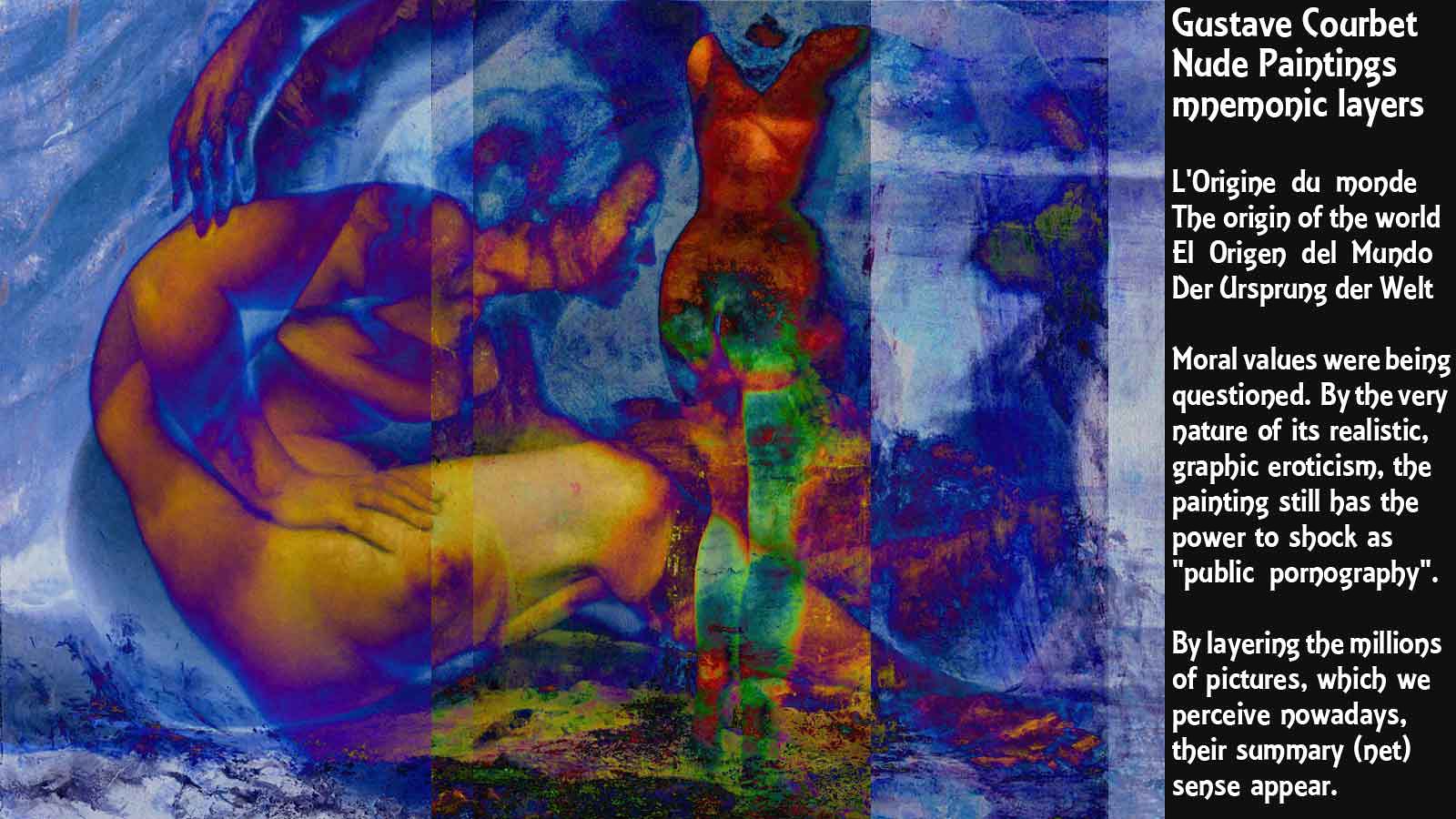The image is a promotional notification or advertisement for an artwork that appears to be a digitally abstract representation. On the left side, the artwork features a fragmented and incongruent depiction of a woman's body and head, set against a blue background with gradient variations and splashes of other colors such as orange, green, red, and yellow. The abstract nature makes it challenging to discern the exact subject, but elements like a hand and parts of the body are visible. On the right side, a black rectangle contains white text that reads: "Gustave Courbet Nude Painting Mnemonic Layers. Les Orines du Monde, the origin of the world, moral values were being questioned by the very nature of its realistic graphic eroticism. The painting still has the power to shock as public pornography. By layering the millions of pictures which we perceive nowadays, their summary net sense appears." The artwork and text collectively address the controversial nature of Courbet's work, highlighting how its explicit realism continues to provoke and challenge moral values.